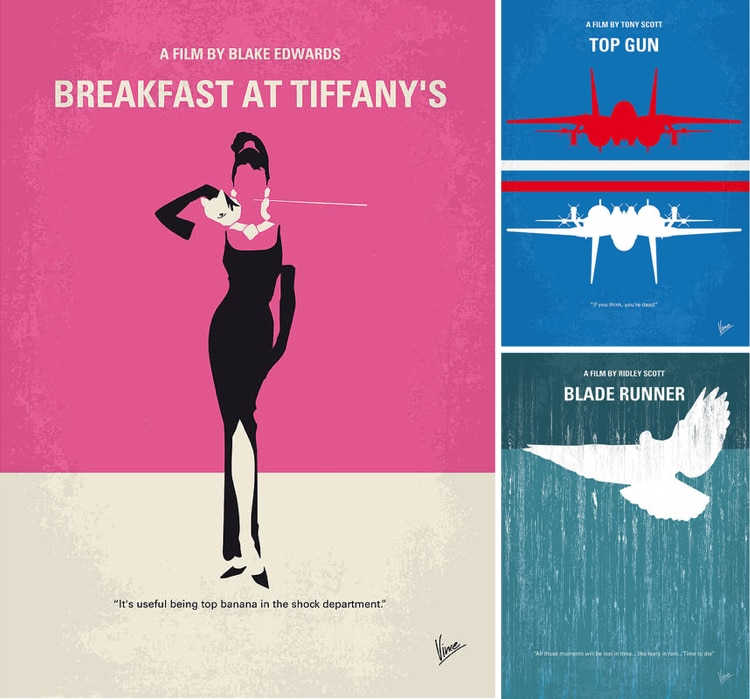Here is a cleaned-up and detailed descriptive caption for the illustrations:

These are artistically reimagined movie posters, each bearing an artist's signature at the bottom.

The first poster, "Breakfast at Tiffany's," created for the 1961 film by Blake Edwards, features a striking figure of a woman against a vibrant pink background. The woman's head is completely pink, while her black hair, accented with pink, is styled up. Adorned with a white diamond necklace and white earrings, she has no facial features, but a long white line extends from where her mouth would be. A black glove encases her hand, and around her neck hangs a white silhouette of a cat. She is dressed elegantly in a black dress paired with black gloves and heels. At the bottom of the poster, in black font, is the phrase, "It's useful being Top Banana in the shock department," accompanied by the artist's black signature.

The second poster, for the 1986 film "Top Gun" by Tony Scott, displays a red plane set against a blue background. Below this, another design features a red line and a white plane, with the title and additional text in white font. The artist’s signature in white is located at the bottom.

The final poster interprets Ridley Scott's 1982 film "Blade Runner" through shades of dark teal and lighter teal. At the top, white font reads, "A film by Ridley Scott." A white bird figure is prominently featured, with additional white text and the artist's signature at the bottom.

Each illustration captures the essence of the respective films while providing a fresh and creative visual take.